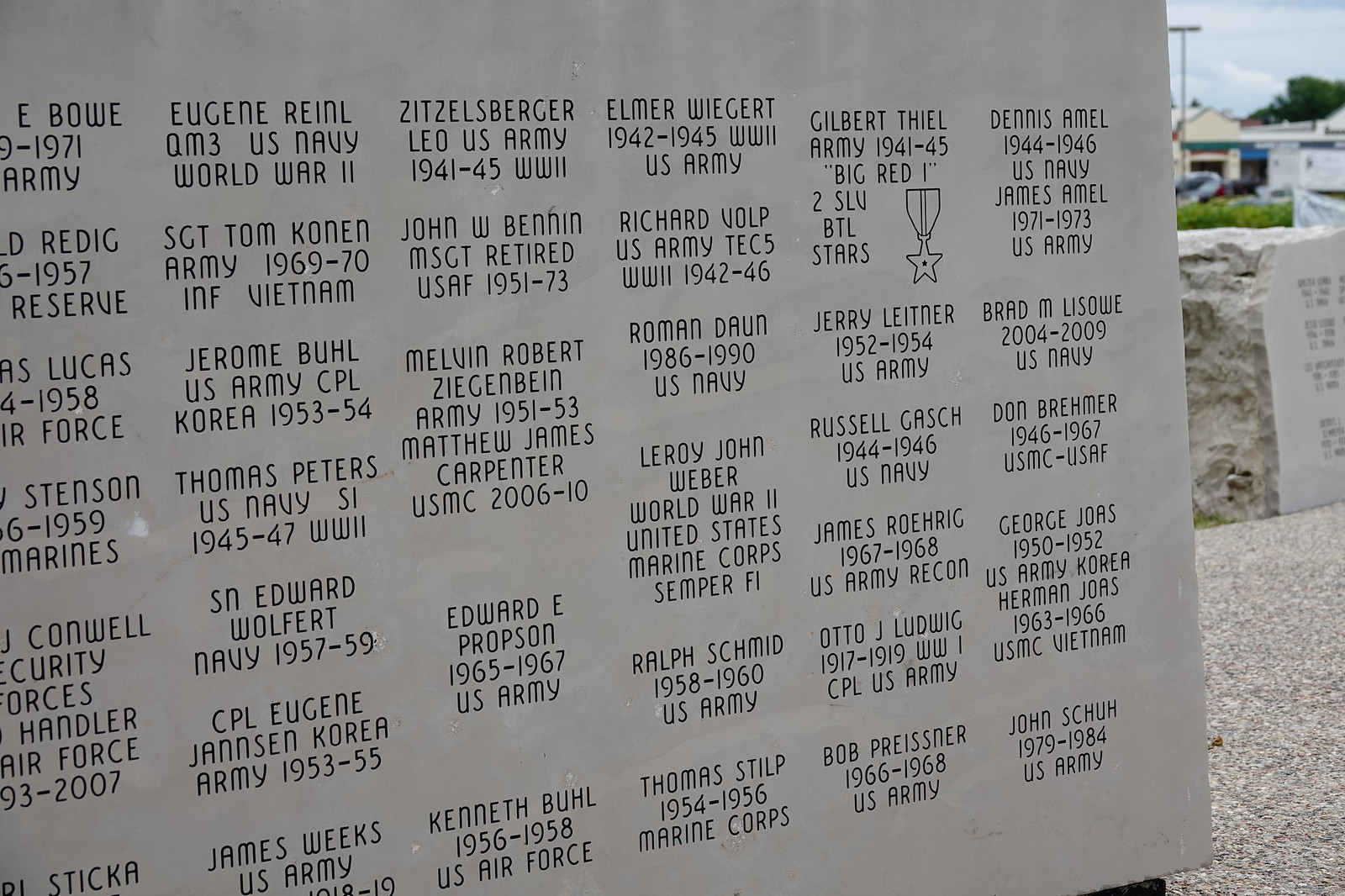The photograph features a light-colored marble memorial plaque, engraved with numerous names of military personnel in dark lettering. The foreground prominently displays this gray stone, organized into roughly six rows and columns of names, though it extends out of the image's frame, suggesting there are many more tributes on this expansive memorial. Among the visible inscriptions are: Eugene Reynold, QM3 U.S. Navy, World War II; Sgt. Tom Conan, Army, 1969-70, INF Vietnam; Jerome Bull, U.S. Army, Corporal, Korea, 1953-54; Thomas Peters, U.S. Navy, S.I. 1945-47, World War II; Essin, Edward Wolfit, Navy, 1957-59, CPL; Eugene Janssen, Korea Army, 1953-55; James Weeks, U.S. Army; Leo Zilbergen, U.S. Army, 1941-45, World War II; and John W. Binghein, MSGT, retired, U.S. AF, 1951-73. Additional names include Melvin Richard, Robert Zingenman, and Dennis Amell, among others. The background reveals additional plaques, a building, sky, and trees, setting the scene in a serene outdoor environment dedicated to commemorating these veterans' service.